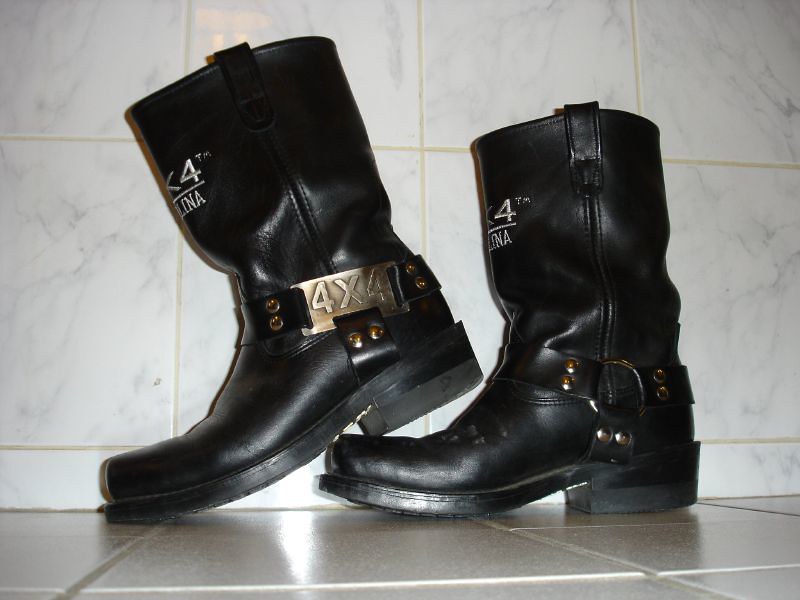In this indoor photograph, two black cowboy boots are placed on a white ceramic tile floor, which also serves as the background, creating a seamless look with slightly darker white grout lines. Both boots have a slight heel and stand nearly above ankle height. The boot on the left has its heel resting on the toe of the boot on the right, with both pairs' toes pointed to the left. Notably, the boots feature distinctive straps: the left boot is equipped with a black strap that includes a gold plate reading "4X4," while the right boot has a similar black strap but adorned with a round, gold-colored ring. Additionally, the front stitching on both boots spells out "4X4" followed by "Carolina" underneath.